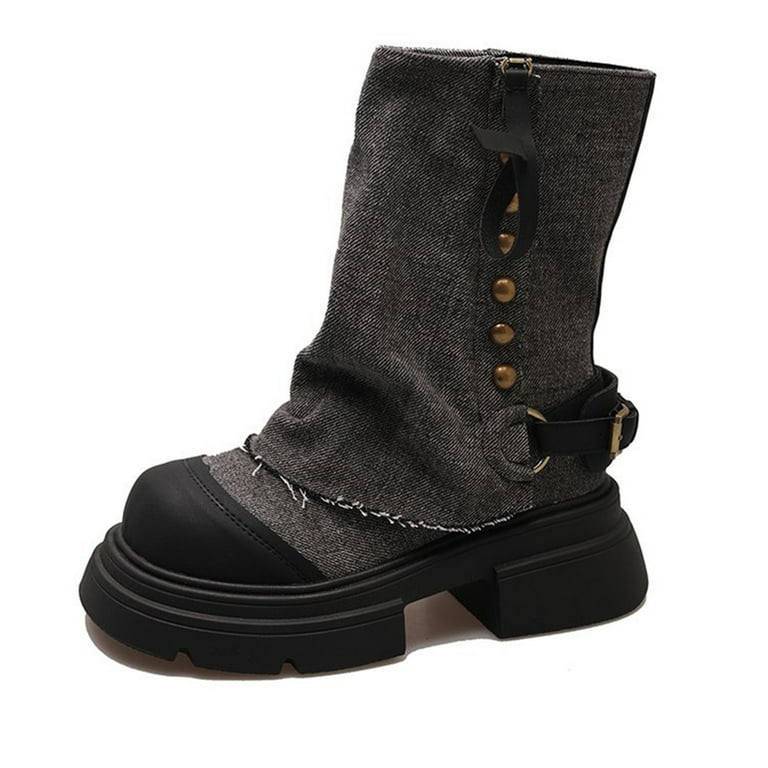This image is a detailed product photo of a stylish boot set against a pristine white background, likely intended for a display ad or digital catalog. The boot, designed to mimic mid-calf height, features a blend of gray and black elements. The upper portion of the boot is made from a dark black leather and possibly dark grey denim that appears slightly frayed. A distinctive feature is the five bronze buttons aligned in a row on the side, adding a touch of rugged elegance. 

The boot incorporates intricate detailing, including a black leather strap that wraps around the heel and another strap connecting to a zipper tab at the top. The toe area is reinforced with a black rubber cover, adding durability. The sole of the boot is particularly noteworthy, being thick and elevated, with a pronounced arch and a substantial heel to provide both style and support. This boot perfectly blends utility with fashion-forward design elements, suited for a variety of looks.